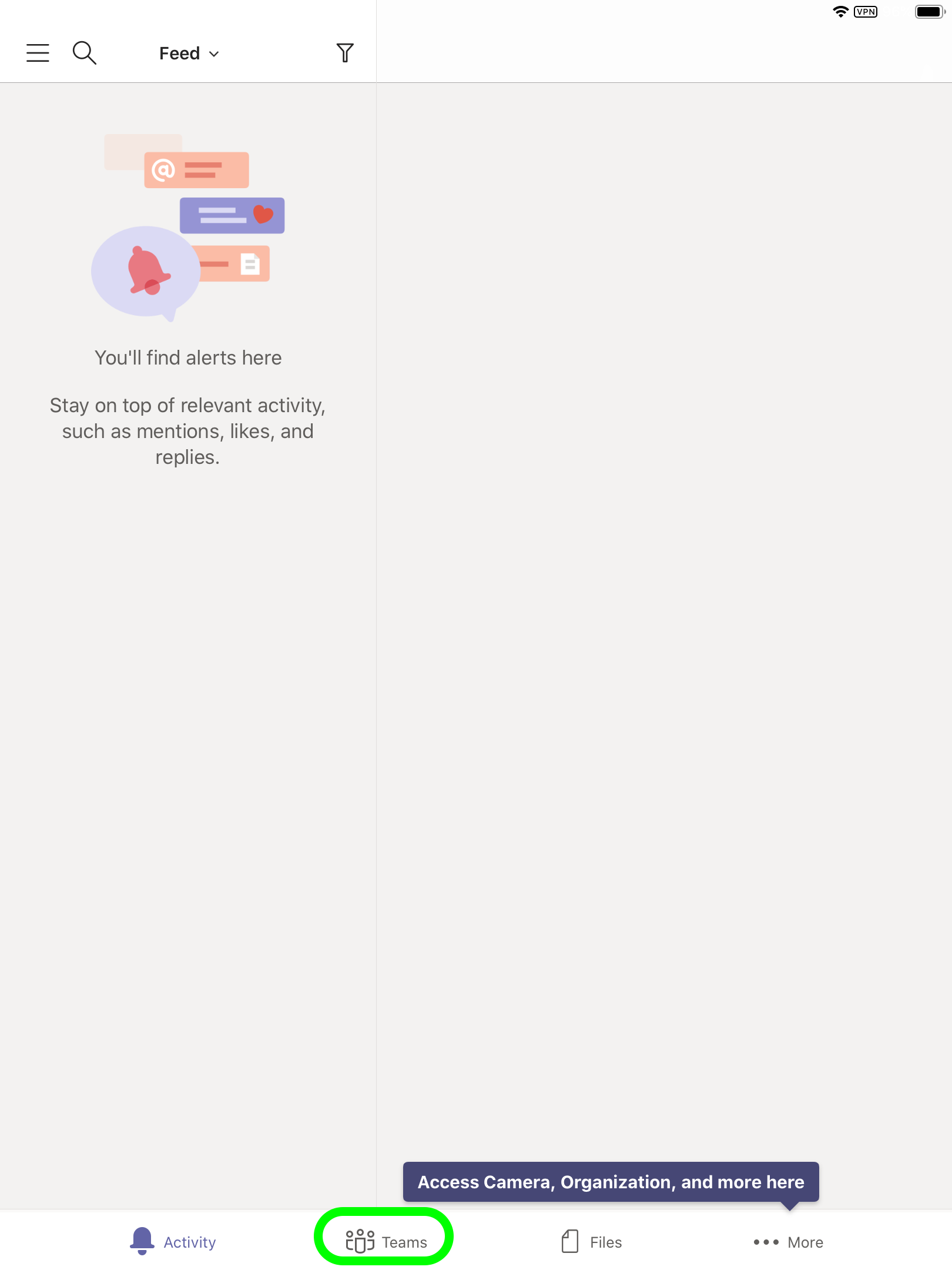This is a detailed screenshot of a social media feed interface captured from a tablet (likely an iPad, as indicated by the horizontal layout). The top left corner features three horizontal lines (menu icon) followed by a magnifying glass icon (search), a label "Feed" with a downward caret arrow (dropdown menu), and a flashlight icon. Directly beneath, there's a message stating, "You'll find alerts here. Stay on top of relevant activities such as mentions, likes, and replies," accompanied by a mini graphic that includes a speech bubble with an alarm bell inside. Additional graphics illustrate various icons: messages, an "@" symbol, a heart symbol, and a document symbol.

At the bottom of the screen are four icons indicating different sections: an activity icon with a bell (representing notifications), a reference to "Teams," a files icon, and a "more" option designated by a triple dot. A speech bubble is displayed above the "more" option, stating, "Access camera, organization, and more here." Notably, the "Teams" icon is circled in green, highlighting its selection.